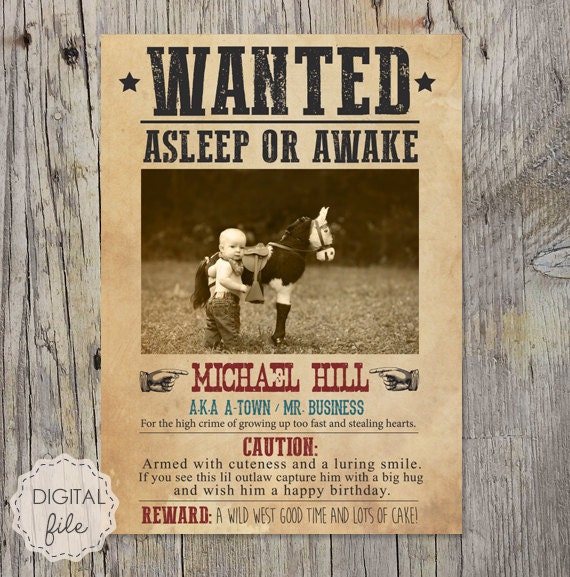This is a color photograph of a custom-made, mock "Wanted" poster mounted on a worn wooden wall, depicting a humorous take on a wild west theme. The poster, designed with an aged sepia tone and bordered by two five-pointed black stars at the top, reads in large black letters "WANTED: Asleep or Awake." Below, a sepia-tone photograph features a toddler named Michael Hill, aka A-Town, Mr. Business, standing next to a toy pony on a lawn. The poster humorously lists his high crimes as "growing up too fast and stealing hearts" and warns that he is "armed with cuteness and a luring smile." It encourages anyone who sees this "little outlaw" to capture him with a big hug and wish him a happy birthday. The final note offers a reward of "a wild west good time and lots of cake." In the bottom left corner, there is a digital watermark in a shield shape indicating the file's digital nature.